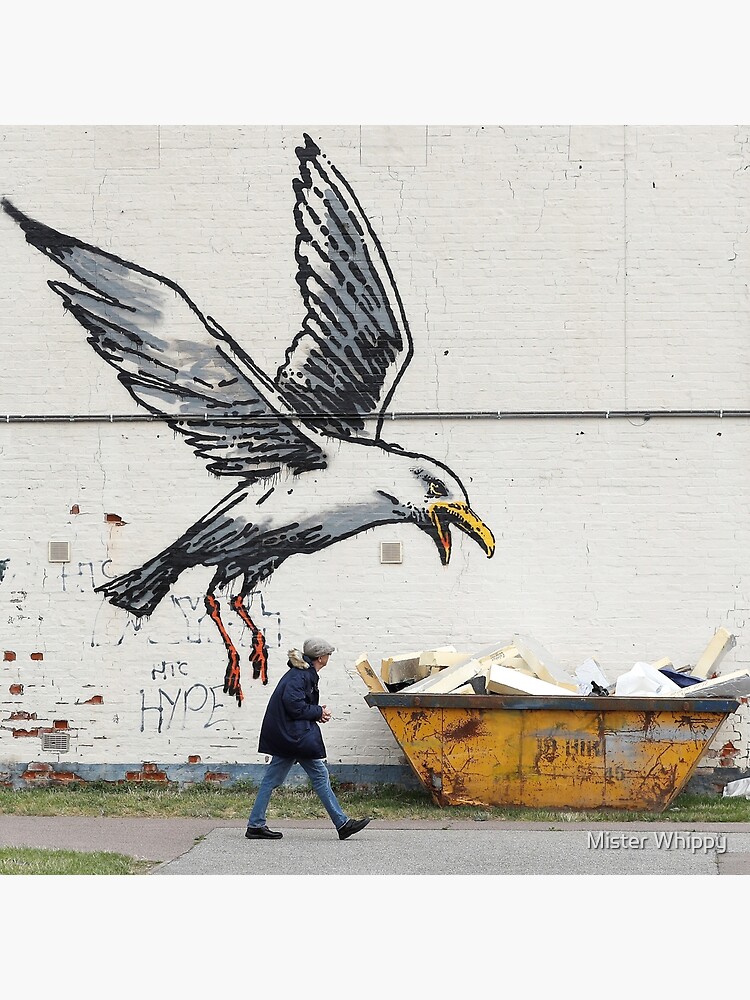The image is a color photograph taken outdoors, depicting a white wall adorned with a large mural of a seagull with outstretched wings. The seagull appears to be swooping down towards a yellow garbage container positioned directly under its beak, giving the illusion that the bird is about to peck at the contents, which include pieces of wood and assorted debris. In the foreground, a man wearing a blue coat, jeans, shoes, and a hat is walking along the sidewalk, glancing up at the mural. The text "Mr. Whippy" is visible in white in the bottom right corner of the image. This scene creates a striking juxtaposition between the whimsical mural and the everyday street activity.